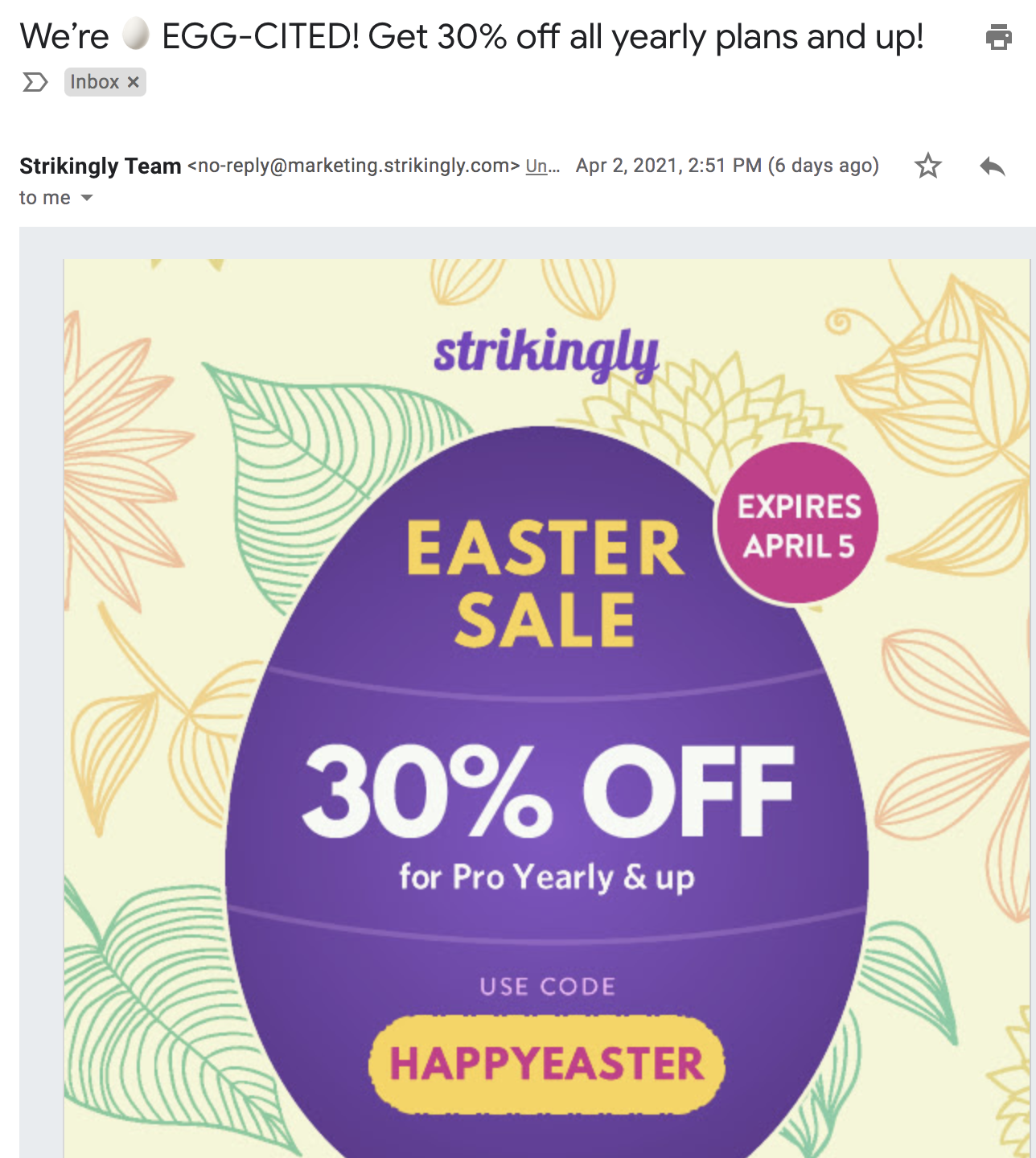Screenshot of an email advertisement in an inbox: 

At the top, there is a white background with black text stating, "We're Eggcited," with an egg emoticon following the word "We're." The word "EGGCITED" is written in all capital letters. The text continues, "Get 30% off all yearly plans and up," ending with a printer icon.

Below this line, there's a right-pointing arrow and an "Inbox" label. The email is from the "Strikingly Team" with the email address "noreply@marketing.strikingly.com." It was sent on April 2, 2021, at 2:51 p.m., which was six days ago.

The advertisement itself features a light blue background overlaid with a beige section adorned with line drawings of floral elements, including leaves and flowers. In the center is a purple Easter egg. At the top of the ad, the word "Strikingly" is written in purple. The main text of the ad states, "Easter sale expires April 5th, 30% off for pro yearly and up. Use code HAPPYEASTER."